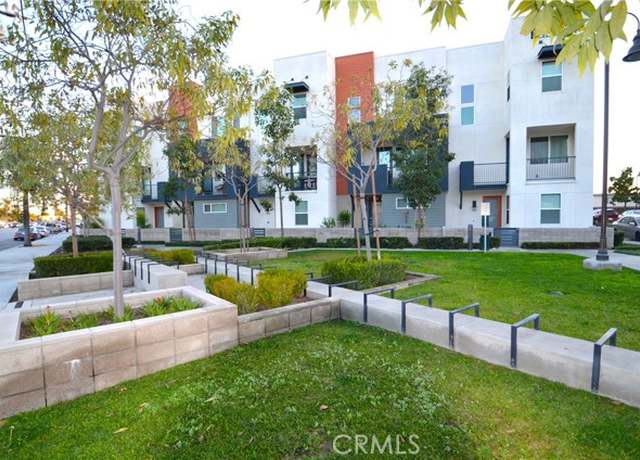The image showcases a modern, multicolored townhouse apartment building with a predominantly white facade, accented by bright red and blue sections. The building's design features several boxy sections, each with its own windows and balconies, though the balconies are empty, leaving it unclear if the building is currently occupied. 

In the foreground, a well-maintained courtyard greets the viewer, consisting of a grassy lawn interspersed with smaller trees and plants set in concrete planters. These planters serve as barriers that lead to a central walkway, merging into a larger sidewalk that connects the building to the street. 

On the far left, a clear sidewalk can be seen, while on the far right, a street light and parallel-parked cars hint at the urban setting. Across the street from the building, other structures are visible, emphasizing the city environment. A parking lot is situated to the right of the contemporary apartment building, completing the urban residential scene.